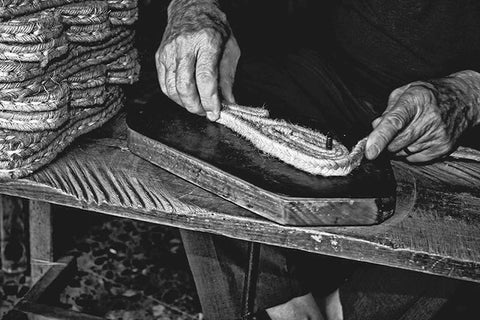In this detailed black and white photograph, an elderly person with wrinkled, liver-spotted hands works meticulously at crafting on a well-worn wooden bench, about waist height, allowing a glimpse of their legs beneath. The individual, dressed in a dark outfit that blends with the bench, appears to be weaving a rug or creating the sole of a shoe using braided rope. This task involves wrapping the rope around pegs that protrude from an oblong wooden object on the bench. In the top left corner of the image, piles of fabric-like materials suggest either a supply of crafting materials or finished products. Their workspace speaks to years of use and the practiced, skilled hands of the elderly artisan add a touching depth to the scene.